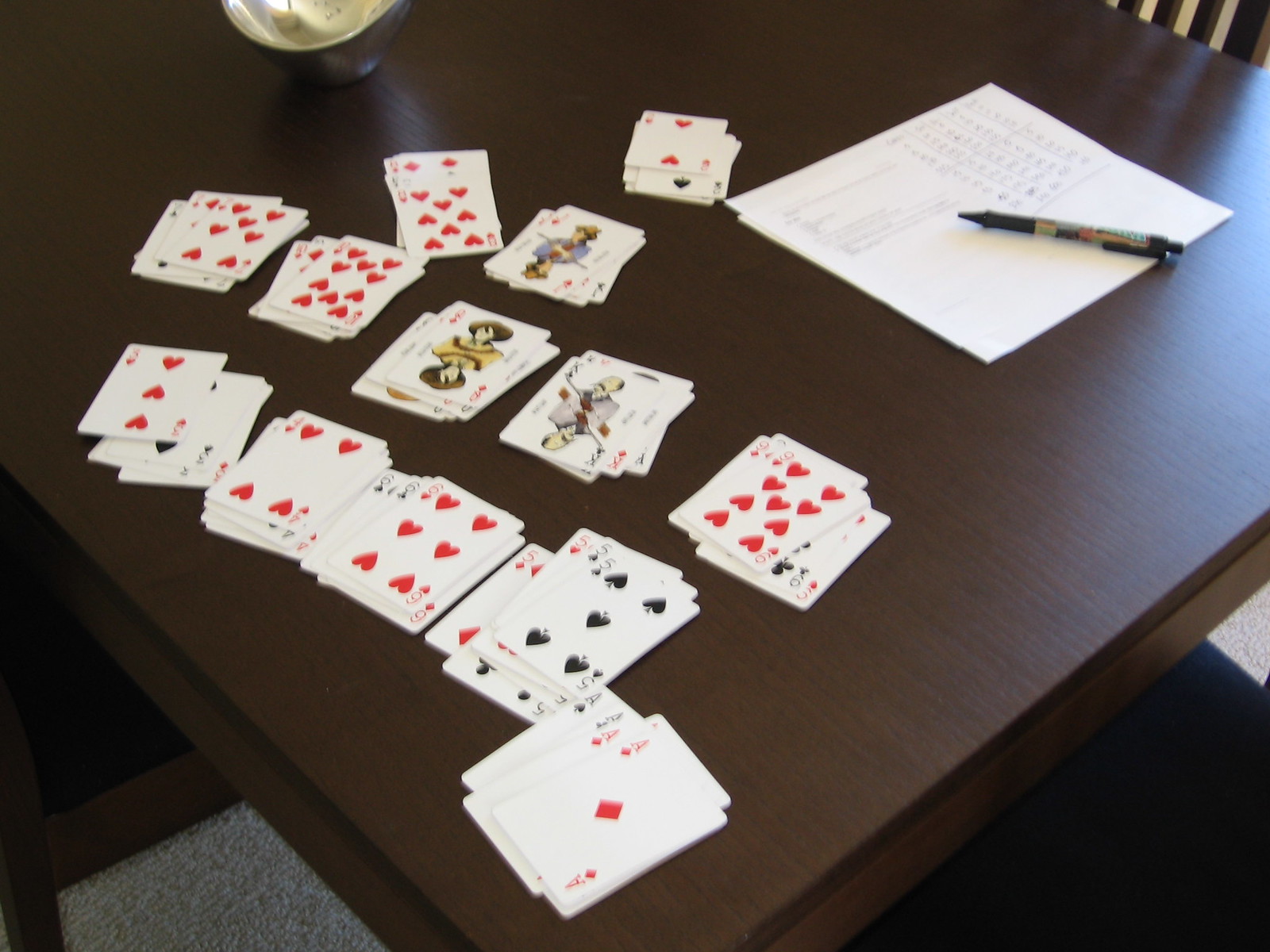In an indoor setting featuring a warm, brown table atop a beige carpet, an array of playing cards is scattered across the tabletop. Positioned at the upper center is a two of hearts, surrounded by a variety of other cards including a jack of diamonds, six of hearts, four of hearts, nine of hearts, three of hearts, another four of hearts, another six of hearts, five of spades, ace of diamonds, and another nine of hearts. In the upper right corner of the table, a piece of paper lies beneath a black ink pen, adding a touch of casual organization to the scene. The image captures a moment of gameplay or card sorting, exuding an inviting and intimate atmosphere.